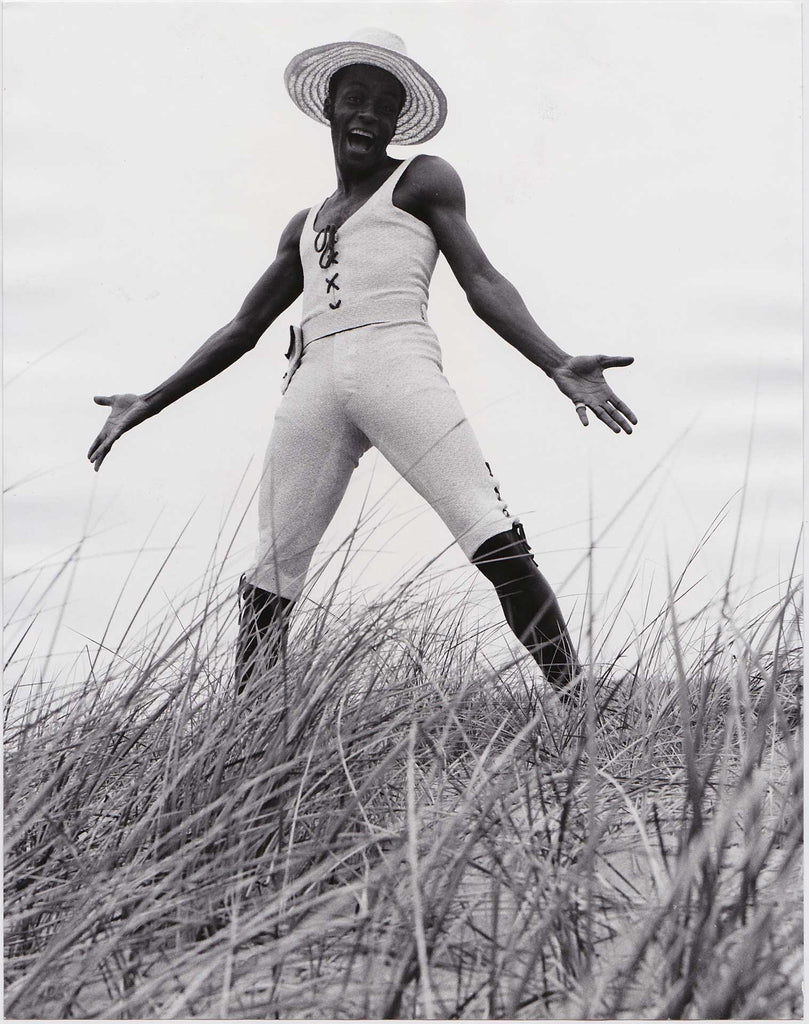In this black and white photograph, a black man stands confidently in a patch of dead grass and brown, dry dirt. His outfit consists of a white tank top featuring unique details such as X's and string marks down the center, along with a bow tie fashioned out of the strings at the top. He is also wearing white shorts that end just below his knees and black knee-high boots. On his head rests a wide-brimmed straw hat, providing a striking contrast to his broad smile. His arms are outstretched with palms forward and fingers splayed, as if striking a joyful pose. The man's face is slightly tilted to the right and downward. Behind him, the sky is a blend of white and gray shades, adding to the image's nostalgic feel. The overall scene evokes a sense of happiness and perhaps hints at a performative moment from an era long past.